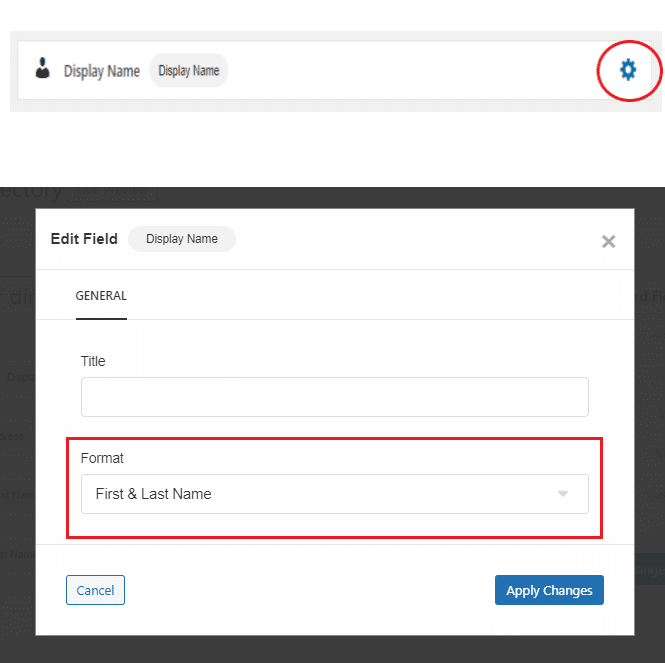In the top section of the interface, outlined in light gray, there is an image of a person's head. To the right of this image, the words "Display Name" appear, followed by the repetition of "Display Name" inside a light gray rectangle. Adjacent to this, a settings icon, resembling a blue wheel, is highlighted with a red circle. Below this, there is a square with a black outline containing information on a white background. In the upper left corner of this square, the word "Edit" is displayed in black. To the right, inside a gray circle, is the text "Display Name." Below this, the word "General" is underlined. The word "Title" appears next, contained within a rectangle, situated above a long rectangle. Additionally, the phrase "Format: First and Last Name" is enclosed within a red rectangle. In the bottom left corner, the word "Cancel" is displayed in a blue rectangle, and finally, in the bottom right corner, "Apply Changes" is written in white text inside another blue rectangle.